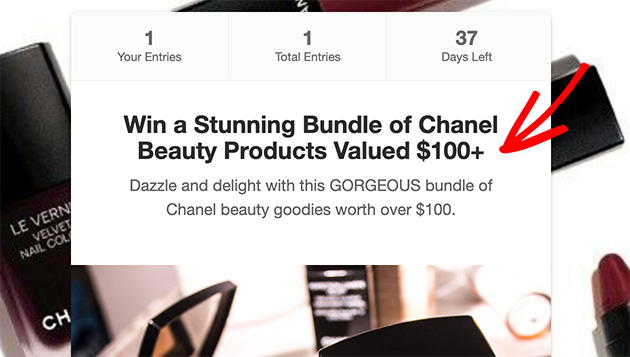Screenshot of a website advertisement showcasing various makeup items, including nail polishes and compacts, arranged on a white surface. In the center, a white square features the text in the upper left corner: "1" with "your entries" below it. To the right, it states "1" with "total entries" below, followed by "37" indicating the total number of entries, with "days left" beneath. Below this section, a line divides the space, with the text "Win a stunning bundle of Chanel beauty products valued at $100+" underneath. Following that, it reads, "Dazzle and delight with this gorgeous bundle of Chanel beauty goodies worth over $100." A photoshopped red arrow points at the "$100+" highlight, drawing attention to the prize's value.